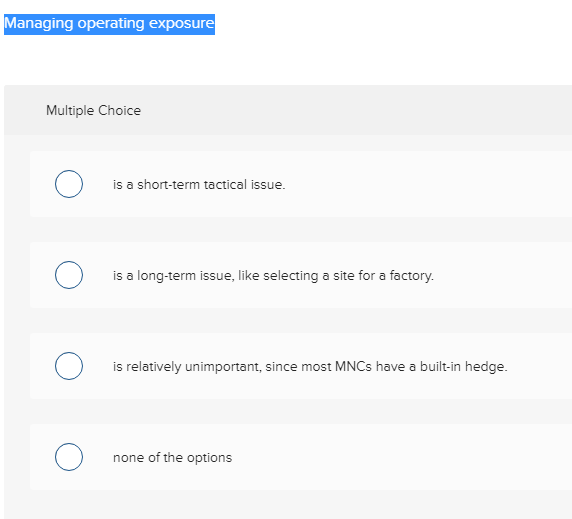The image depicts a multiple-choice question likely sourced from a quiz or test. The header at the top reads "Multiple-Choice" in a very thin, black sans-serif font against a light to medium gray background. The text in the header appears blurry, hinting at the poor image quality.

Above the multiple-choice section, there is a highlighted area which states "managing operating exposure". The text here is white, situated on a blue-highlighted backdrop.

The multiple-choice options are presented as follows:

1. "Is a short-term tactical issue."
2. "Is a long-term issue, like selecting a site for a factory."
3. "Is relatively unimportant, since most capital MNCs have a built-in hedge."
4. "None of the options."

Each option is enclosed in a very light gray rectangle with black text in the same basic sans-serif font as the header. The selection circles next to each option are white with a dark blue border, and none of them are filled in or checked. This indicates that no answer has been selected.